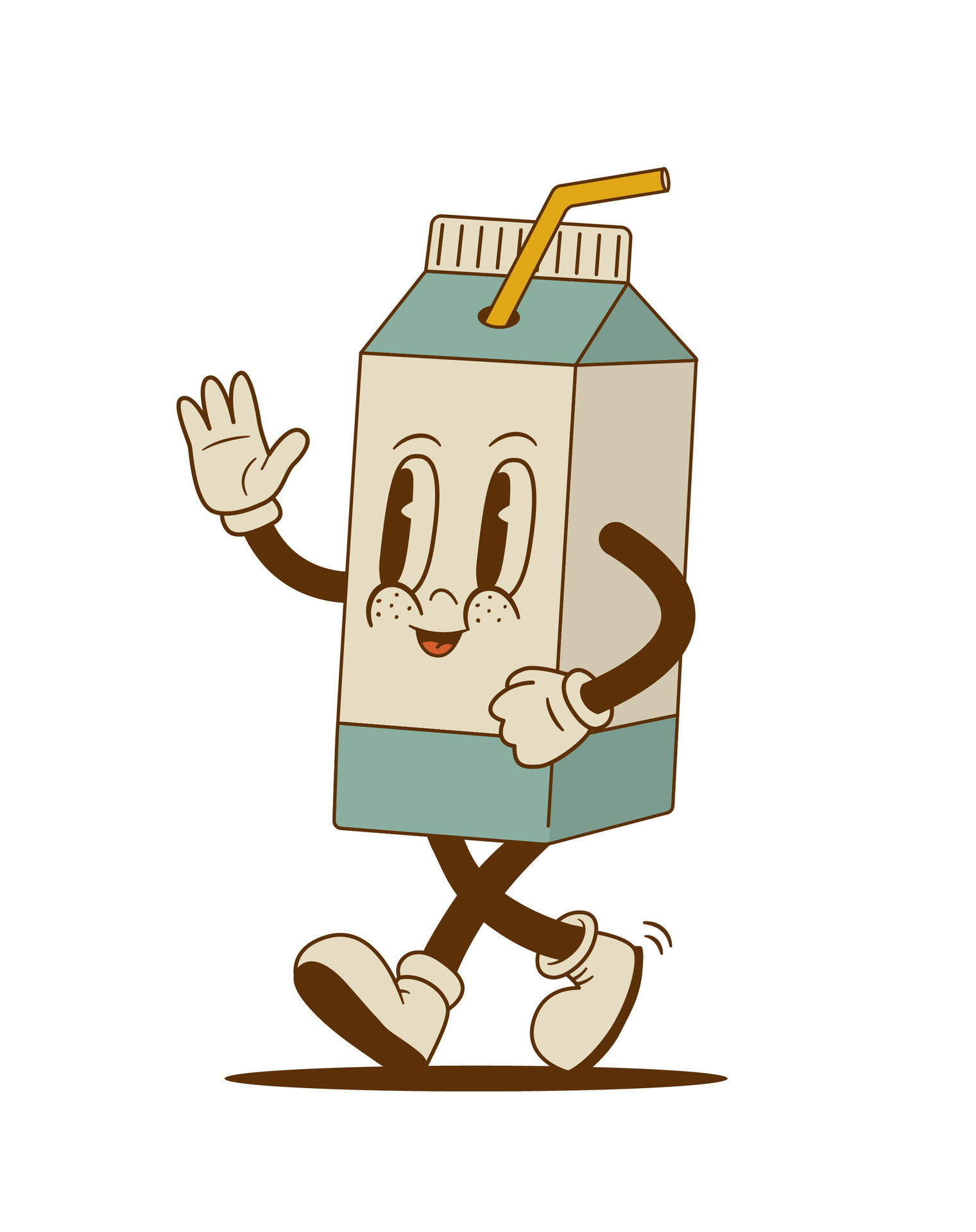The image depicts a whimsical, anthropomorphized milk carton set against a pure white background. The white and blue carton boasts a triangular roof with an orange straw emerging from a hole at the front and bending to the right. The carton features a cheerful face with large, oval-shaped brown eyes, red cheeks, and a smiling mouth showing a pink tongue. Its body is rectangular, with two bendable, brown arms ending in white gloves, reminiscent of classic cartoon characters. The right arm is raised in a friendly wave, with the gloved hand's palm facing forward, while the left arm hangs downward. The bottom of the carton has a green border and two legs, similar in style to the arms, each wearing brown or beige shoes. A subtle shadow beneath the carton adds a sense of dimension and movement, suggesting the character is walking towards the left side of the frame.